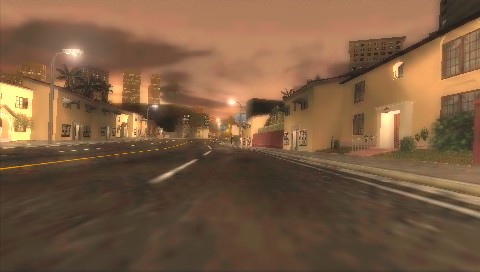This blurred photograph seems to have been taken from a moving vehicle at twilight or nighttime. The scene captures a quiet asphalt road flanked by sidewalks, illuminated by streetlights. On both sides of the road stand uniformly designed, cream-colored, flat-roofed buildings that resemble a resort area, possibly built with stucco. Some minimal landscaping is visible in front of the structures, adding to the ambiance. Majestic palm trees rise behind these buildings, creating a tropical atmosphere. In the background, the silhouette of lit-up skyscrapers looms, indicating an urban environment nearby. Down the empty road, more streetlights dot the scene, contributing to the serene, almost eerie, quietness. The sky above is a blend of pinkish-gray hues, with clouds scattered across, enhancing the overall dreamy mood of the photograph.